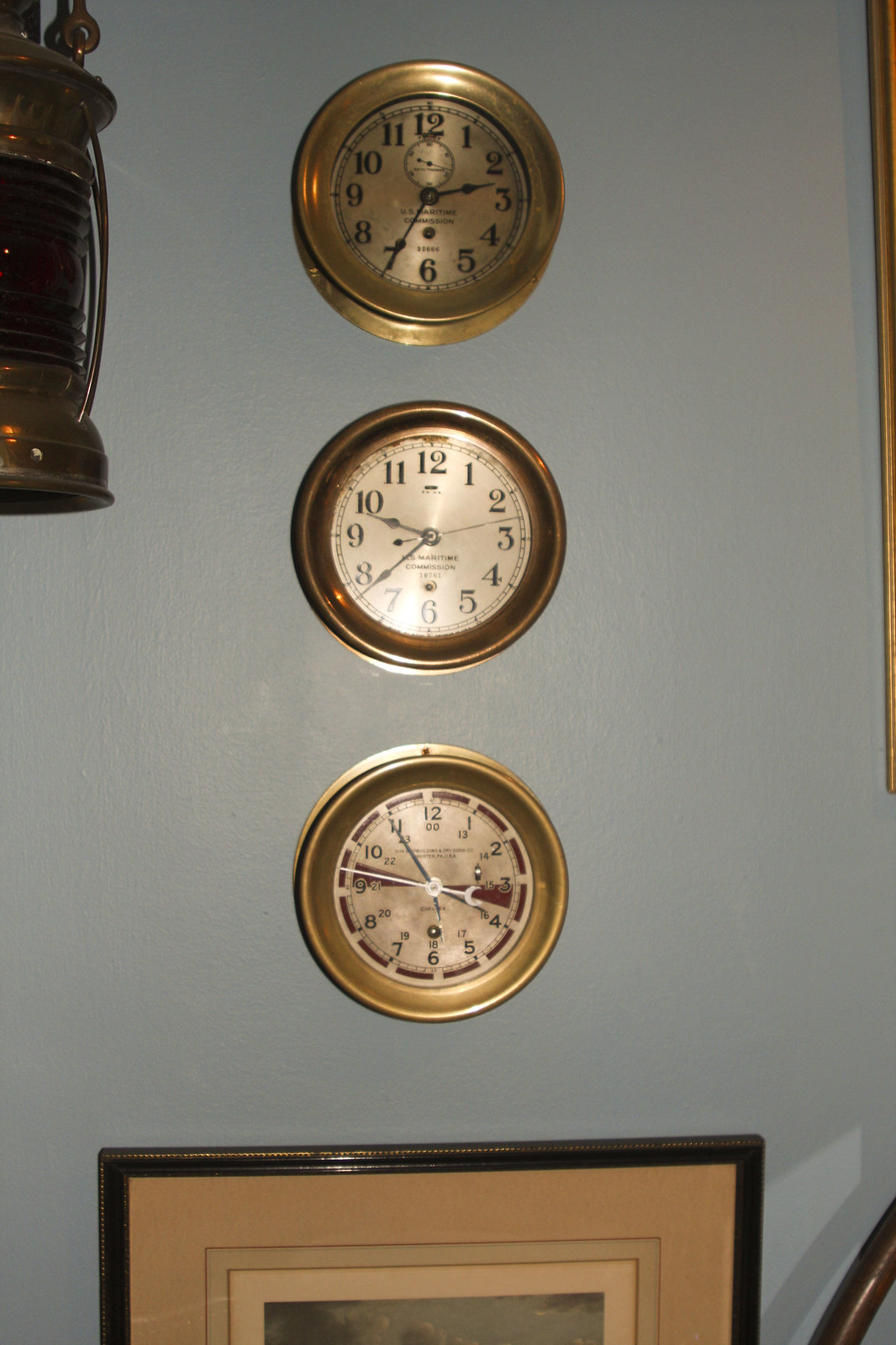The photograph captures a rectangular scene featuring three circular wall clocks mounted on a light blue wall. The left and right sides of the image are notably longer than the top and bottom edges. In the lower portion of the image, a brown ornate frame containing a tan-colored border surrounds a painting, which is mostly out of view to the left. Adjacent to this painting on the right is a wooden stair railing.

Above these elements on the wall are the three clocks, all sharing similar designs with brass frames encircling silver clock faces. Despite the cohesive aesthetic, each clock possesses slight variations in their markings and styles. The top clock prominently displays bold black numbers, with small squares marking the minutes between each numeral. This clock currently reads 2:35, showcasing a meticulous blend of utility and decorative charm. The detailed arrangement of these elements brings a balanced, vintage feel to the composition.